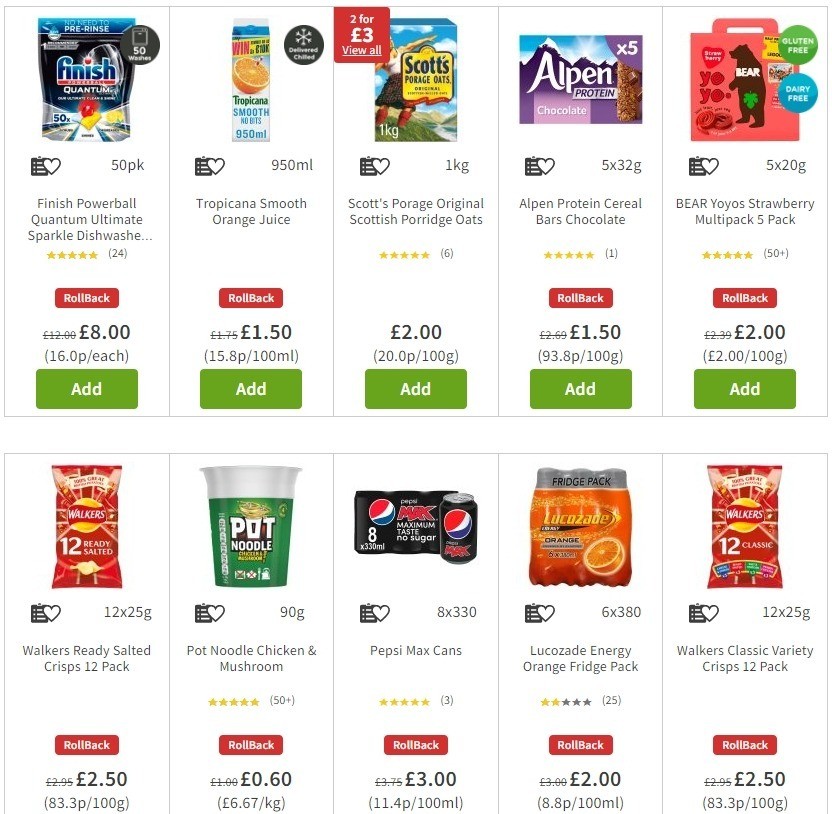The image features a white background showcasing ten distinct products, complete with price reductions and interactive elements. Here's a detailed breakdown of each product:

1. **Finish Powerball Quantum Ultimate Sparkle Dishwashing Liquid**:
   - Highlighted with a black star.
   - Priced at $8 with a rollback indicator in red.
   - Includes a green "Add" button.
   
2. **Tropicana Smooth Orange Juice**:
   - Features a black heart icon.
   - Rollback price of $1.50, highlighted in red.
   - Includes a green "Add" button.
   - In the upper left corner, there's a red box indicating a promotion: "2 for $3, view all".

3. **Scots Porridge Original Scottish Porridge Oats**:
   - Displayed with a black heart icon.
   - Priced at $2.
   - Includes a green "Add" button.

4. **Alpen Protein Cereal Bars Chocolate**:
   - Accompanied by a black heart icon.
   - Rated five stars.
   - Rollback price of $1.50, highlighted in red.
   - Includes a green "Add" button.

5. **Bear Yo-Yo Strawberry Multipack (5 pack)**:
   - Features a black heart icon.
   - Rated five stars.
   - Rollback price of $2, highlighted in red.
   - Includes a green "Add" button.

6. **Walker's Ready Salted Crisps (12 pack)**:
   - Highlighted with a black heart icon.
   - Rollback price of $2.50, highlighted in red.
   - Includes a green "Add" button.

7. **Pot Noodle Chicken and Mushroom**:
   - Rated five stars.
   - Features a black heart icon.
   - Rollback price of $0.60, highlighted in red.
   - Includes a green "Add" button.

8. **Pepsi Max Cans**:
   - Features a black heart icon.
   - Rollback price of $3, highlighted in red.
   - Includes a green "Add" button.

9. **Lucozade Energy Orange Fridge Pack**:
   - Highlighted with a black heart icon.
   - Rollback price of $2, highlighted in red.
   - Includes a green "Add" button.

10. **Walker's Classic Variety Crisps (12 pack)**:
    - Features a black heart icon.
    - Rollback price of $2.50, highlighted in red.
    - Includes a green "Add" button.

Each product is clearly showcased with its respective price, rating, and promotional details, set against a clean white background for easy visibility.